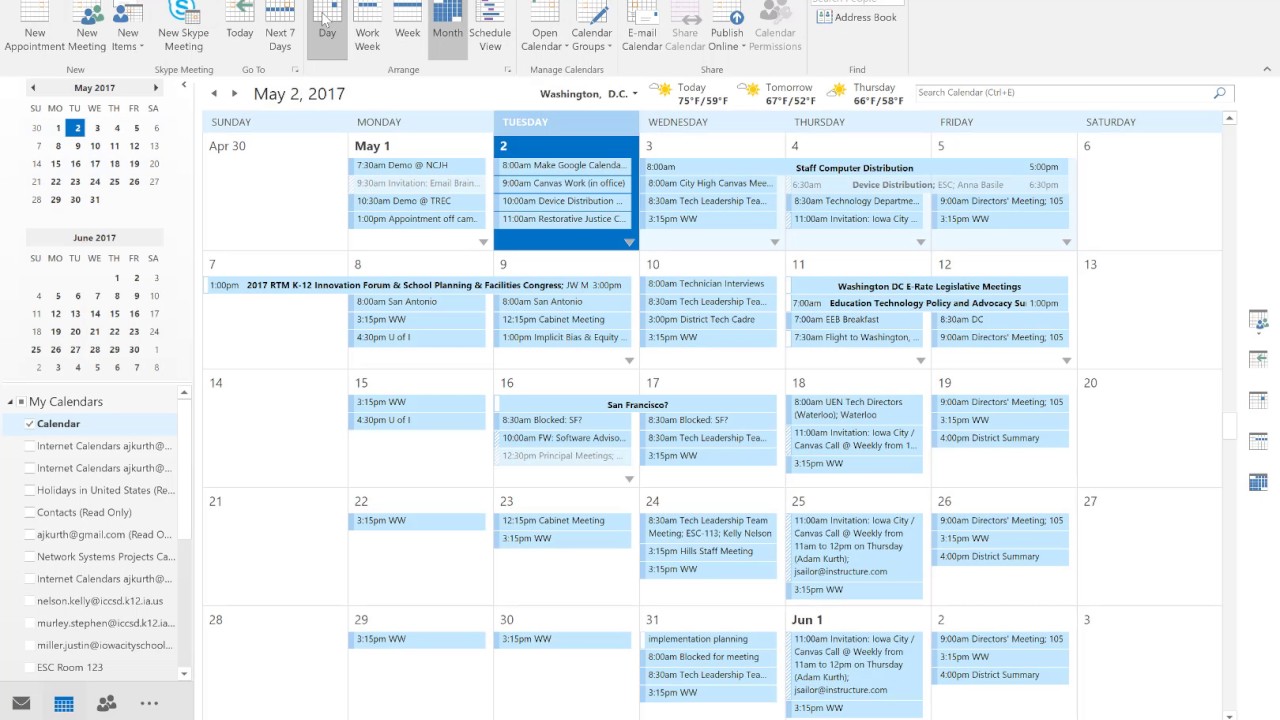The image depicts a detailed spreadsheet interface featuring a calendar for May 2017, specifically from Washington D.C. The weather forecasts are indicated for a few days: today's high is 75°F with a low of 49°F, tomorrow's forecast shows a high of 67°F and a low of 52°F, and Tuesday's projection includes a high of 66°F and a low of 58°F.

At the top center of the spreadsheet, several tables are displayed. The upper section of the interface features buttons for various application functions. The primary section of the screen showcases a calendar populated with scheduled events, focusing on the month of May 2017.

The calendar highlights scheduled dates in blue and lists details in black text. Specific scheduled periods include:
- May 1 to May 5
- May 1 to May 7
- May 1 to May 12
- May 15 to May 19
- May 22 to May 26
- May 29 to June 2

Notably, no events are scheduled for Saturdays, and only one event is set for Sunday, May 7. The calendar event for May 1 is scheduled to start at 7 a.m.